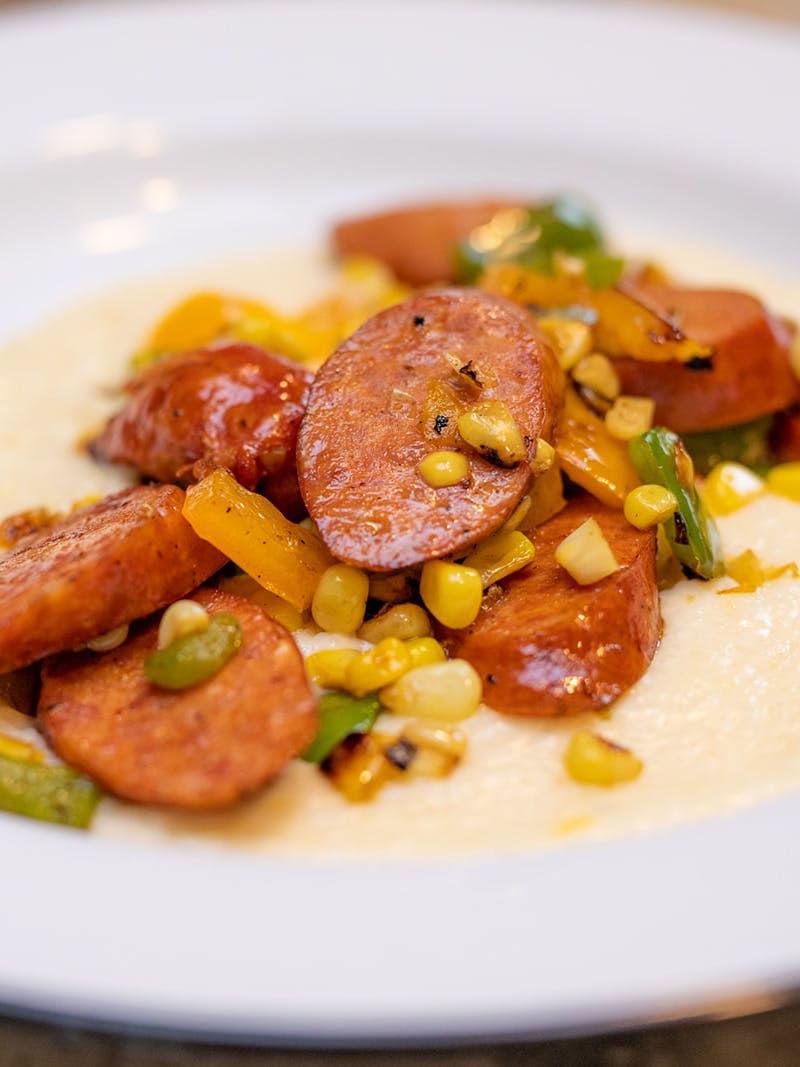This is a close-up image of a meticulously plated dish on a white, slightly depressed plate that is neither completely flat nor a full bowl. At the base of the dish lies a thick, off-white sauce, creating a creamy bed for the other ingredients. Resting atop the sauce are large, shiny slices of reddish-brown sausage, which look freshly fried and glistening as if just out of the skillet. Scattered around the sausage are sautéed corn kernels and yellow bell pepper slices, adding a burst of color. Additionally, chopped green vegetables, likely bell pepper and scallions, are interspersed throughout the mix. The image has high resolution on the focal point—the sausage and vegetables—against a slightly blurred background and plate edges, drawing attention to the fine details of the ingredients.